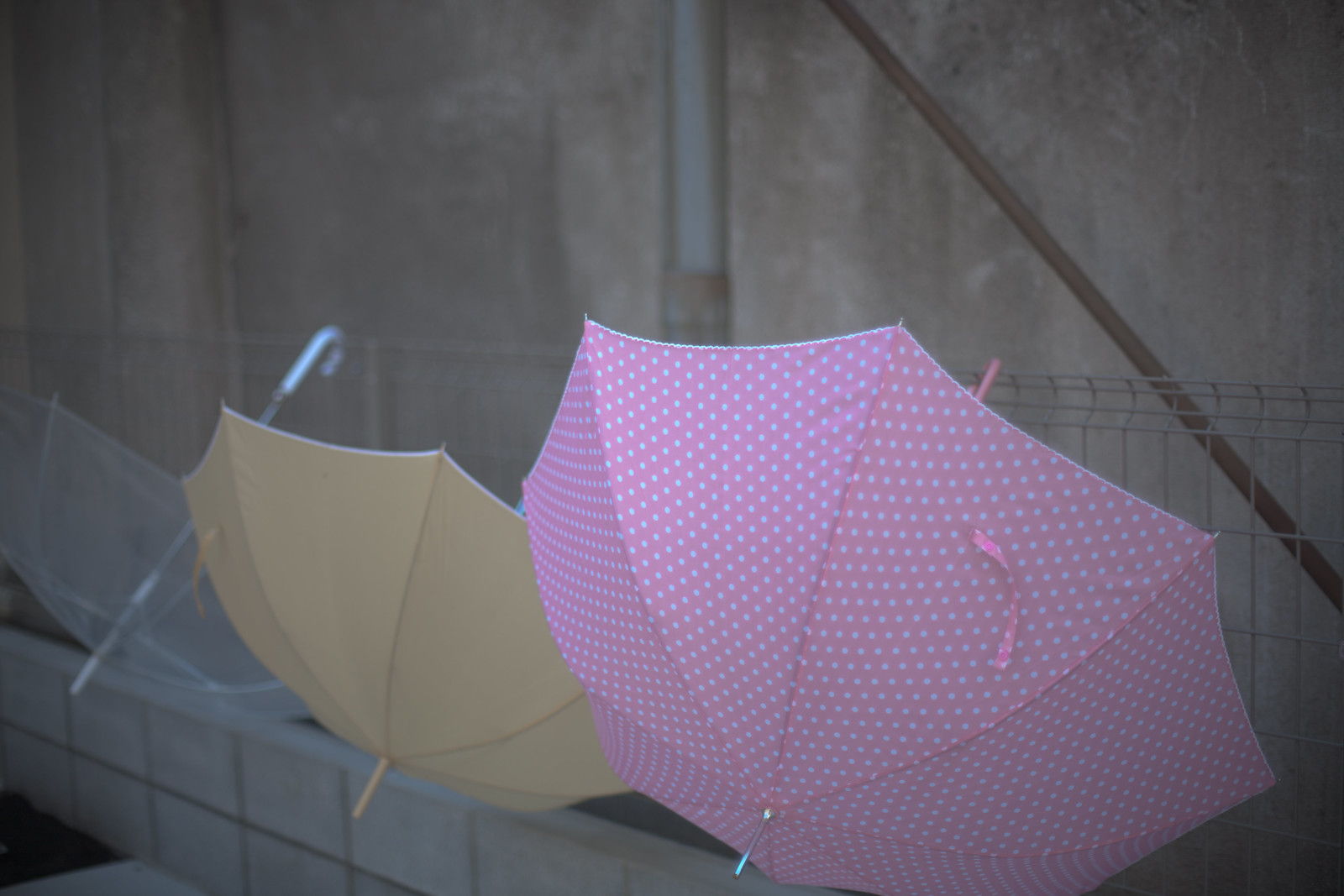This digital photograph captures three open umbrellas hanging on a wire mesh fence, set against a stark gray concrete wall. The wall features a darker gray diagonal pipe running from the right-hand side about a quarter of the way down and a vertical gray pipe in the center. The umbrellas are displayed facing down towards the bottom right of the image. The one closest to the viewer on the right is pink with white polka dots and has a matching white handle. The middle umbrella is a solid light yellow with a white border and yellow spoke emanating from the top. The umbrella on the far left is made of clear plastic, supported by a silver metal pole with a white handle. Below the wire fence, a narrow strip of bare concrete sits above a small patch of either dirt or grass. The scene combines a mix of practical, utilitarian elements with a touch of whimsy from the brightly colored and patterned umbrellas.